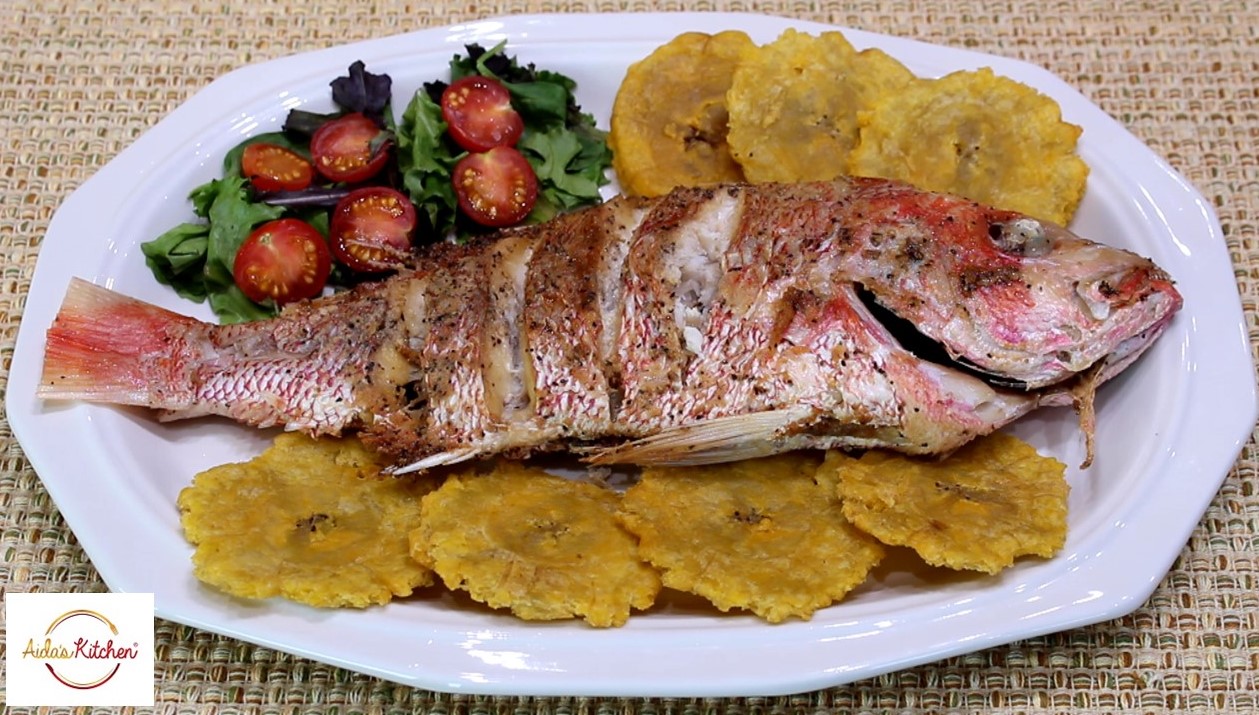In this wide rectangular image, a visually appealing dish is presented on a square white plate bearing a subtle stripe pattern. At the center lies a whole cooked red snapper, its reddish-brown body sporting char marks from grilling and four vertical cuts along its side. The fish retains its head, bottom fin, and tail fin, with its eye missing, revealing it has been gutted and prepared with skill.

Surrounding the fish, there are four slices of fried, flattened plantains neatly arranged at the bottom of the plate, and three more pieces placed at the top right. In the top left corner of the plate sits a small salad of dark mixed greens and six halved cherry tomatoes, their cut sides facing forward, adding a vibrant splash of color to the dish.

Beneath the plate, the setting features a finely woven wicker-like placemat in a cream hue that complements the composition. In the bottom left corner of the image, there is a small, off-white rectangular label with red and yellow text displaying "Ada's Kitchen," adorned with a half-circle design above and below the text, contributing a touch of branding to this culinary presentation.